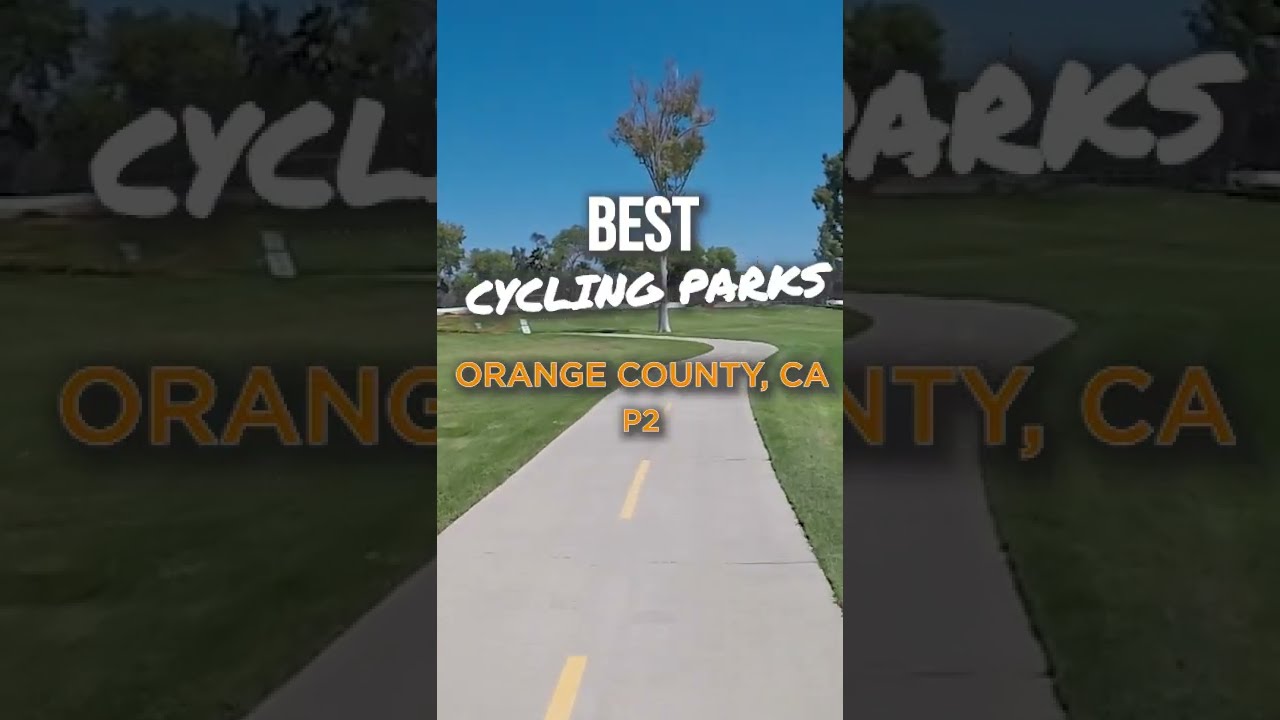The image is a digitally enhanced photograph, resembling a possible snapshot or screenshot from a website or video, featuring the title "Best Cycling Parks" in white text at the top center. Directly below, in orange text, it states "Orange County, CA" followed by "P2." The scene depicts a cycling trail, characterized by a gray path with yellow dashed lines dividing two lanes. The road begins in the middle of the image, curves gently to the right before making a prominent loop to the left. Surrounding the trail is flat, vibrant green grass with a solitary tree in the foreground and additional trees in the background, all under a clear, bright blue sky without clouds. The image is cropped such that no website address is visible, and the outer edges feature a wide border made from grayed-out, magnified elements of the central photo, seamlessly blending into the overall composition. Notably, the scene is devoid of cars, emphasizing the serene, park-like atmosphere of the cycling path in Orange County, California.